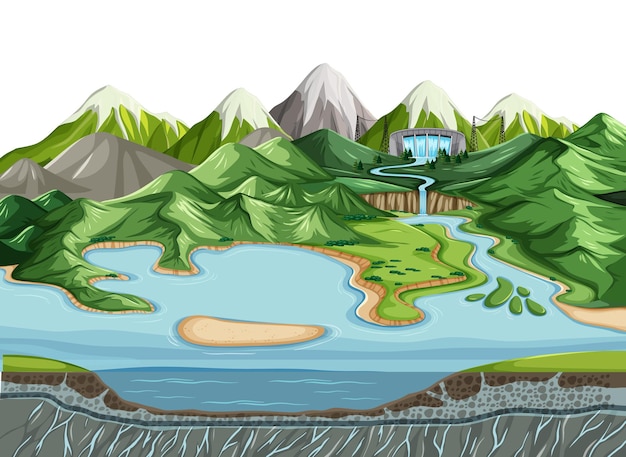This artistic rendering illustrates a comprehensive depiction of the water cycle, seamlessly integrating natural and man-made elements. In the background, majestic snow-capped mountains descend gracefully into verdant foothills, eventually leading to a tranquil lake. The artwork provides a cut-away view of the earth beneath the lake, revealing intricate layers of aquifers and stone strata that facilitate water seepage and storage.

Amidst the mountains, a dam stands prominently, with electric lines extending from it, symbolizing the generation of hydroelectric power. This sustainable energy is harnessed from the meltwater cascading down from the snowy peaks with tremendous force. The water is then channeled into a controlled river, which meanders through the landscape before plunging over a picturesque waterfall and finally feeding into the serene lake.

The lake serves multiple purposes: it is a site for recreation, a reservoir for potable water, and a crucial component of the subterranean water table. Overall, this detailed illustration provides a vivid and insightful portrayal of how water flows through various stages of the hydrological cycle, highlighting both its natural beauty and its pivotal role in human infrastructure.